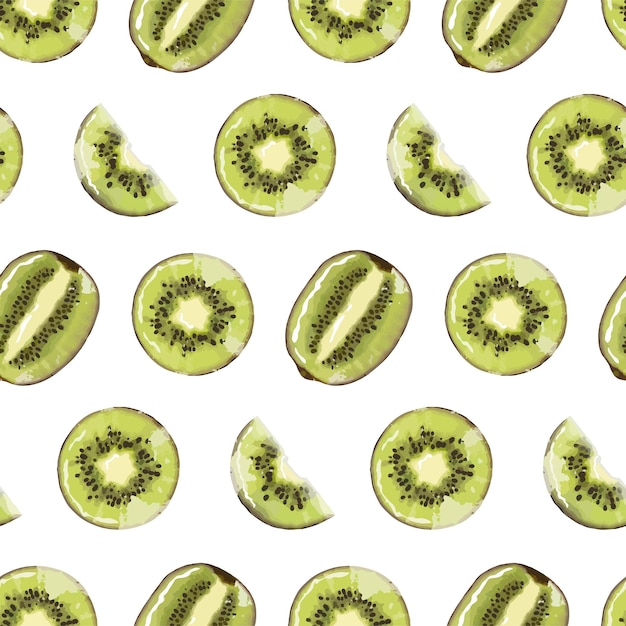This detailed piece of artwork or print prominently showcases kiwifruits arranged in meticulously organized patterns. The kiwifruits are aligned in precise rows both horizontally and diagonally, creating a striking visual symmetry.

In the most distinctive rows, the kiwifruits are sliced horizontally across their thinnest side, revealing circular cross-sections. These slices beautifully display the dark green, slightly fuzzy outer skin, a pale green inner layer encircling tiny black seeds, and the vibrant bright green flesh at the center. These circular slices are alternated with rows featuring the same fruit halves, creating half-moon shapes that offer a contrasting yet harmonious pattern.

Another captivating element of this artwork is the inclusion of kiwifruits cut lengthwise from top to bottom. These sections reveal an elongated oval shape with the familiar dark green outer skin. Inside, a long, thin pale green oval houses the characteristic black seeds, surrounded by the vivid bright green flesh, completing the ensemble.

Together, these varying cuts of kiwifruit, arranged in an intricate blend of symmetry and natural beauty, create a vivid and visually appealing composition that celebrates the unique textures and colors of the fruit.